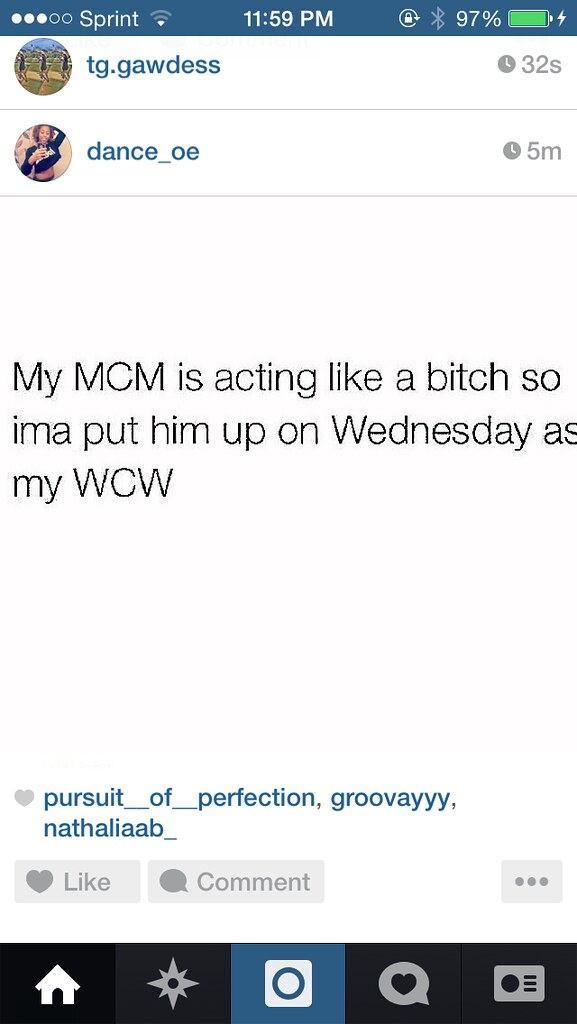The image is a detailed screenshot taken from a cell phone displaying a social media post. It shows a text post from the username "pursuit_of_perfection" with a caption that reads: "My MCM is acting like a bitch so I'ma put him up on Wednesday as my WCW." The screen indicates a Sprint network with only one bar of reception and a battery life of 97%, captured at 11:59 p.m. Additionally, there's an icon next to the handle "tg.goddess," which was active 32 seconds ago, and another next to "dance_oe," active five minutes ago. At the bottom, the username "Pursuit of Perfection" appears along with options for navigating to the home screen, sharing the post, or accessing personal information.